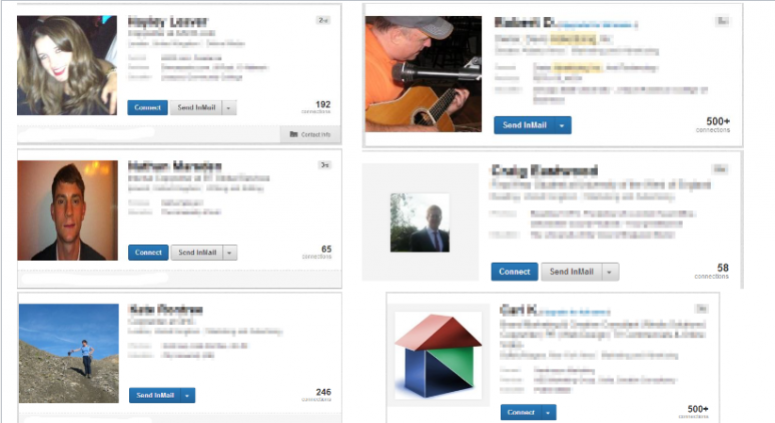Here is a detailed and refined caption for the image:

"This image is an extremely blurred screenshot of what appears to be a LinkedIn webpage, featuring six individually outlined profile blocks arranged in two columns and three rows against a white background. The top left profile depicts a woman with brown hair facing left, accompanied by her name and additional professional details, though these are indistinct. Beneath her name are options to 'Connect' and 'Send a message,' indicative of LinkedIn's interface. To her right is a blurred profile of a man playing a guitar, also showing his name and '500+ connections.'

In the second row, the left profile features a young man who is staring straight at the viewer, along with the 'Connect' option. Adjacent to him, on the right, is a profile with a very small image of a man in a suit, including his name and the 'Connect' button.

The bottom row's left profile showcases someone near the sea, while the bottom right profile displays an image of a house constructed from geometric shapes: a blue triangle, a green triangle, and a red triangle, with associated profile information next to it."